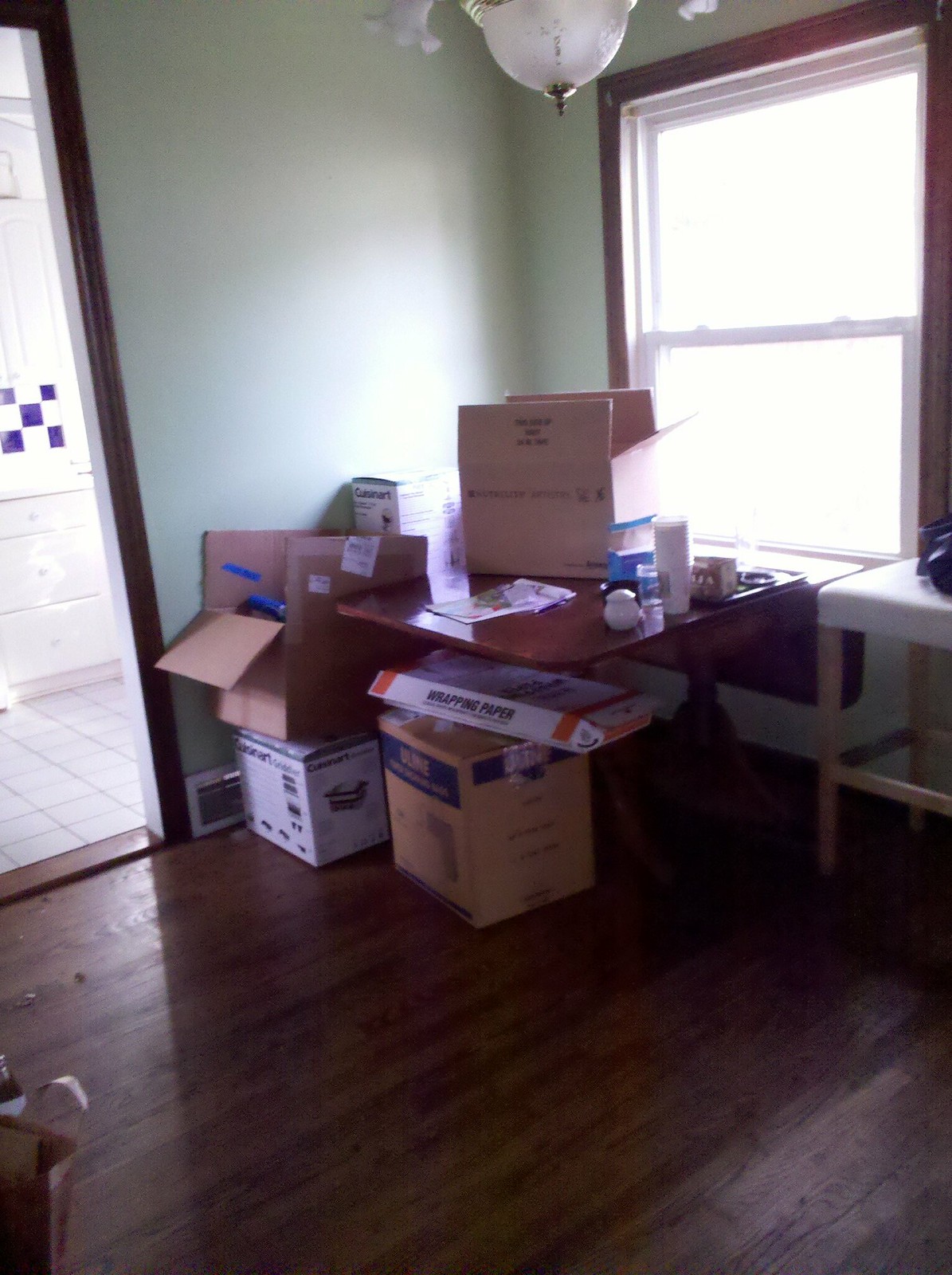This image captures a cluttered corner of a room, possibly within a house or an office. The scene centers on a collection of cardboard boxes, some stacked haphazardly on the wooden floor and others precariously placed. Dominating the corner is a simple wooden table, dark brown in color, holding at least one of these boxes. The table also supports various miscellaneous items, including a plastic bag and what appears to be a stack of cups.

To the right of the wooden table stands a white plastic table, which holds an unidentified black object. A large window occupies part of this corner, allowing an intense flood of natural light to pour in, though it's too bright to reveal the view outside.

The walls of this corner are painted a light green hue, lending a soft, tranquil vibe to the space. Below, the wooden flooring adds warmth to the room. Overhead, a light fixture attached to the ceiling consists of a central glass dome and an adjoining part, likely designed for an additional single light bulb.